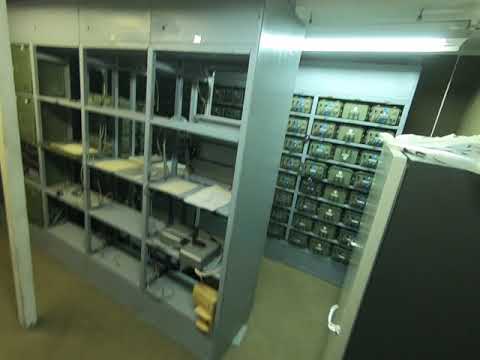The image depicts an industrial room with a concrete floor and a white-painted steel beam rising on the left side. The focal point is a series of gray metallic shelves, viewed from a height similar to a security camera perspective. The shelves are divided into four rows and columns, with sparse contents. The top shelf contains several organized papers, and the shelf below it holds a few smaller items. Notably, there are green boxes neatly arranged in columns and rows on the top shelf at the back. The room is illuminated by a fluorescent light running horizontally across the top. To the right of the shelves, there's a cabinet with a dark gray body and an off-white door, featuring a chrome handle. The wall behind the shelves is also gray and adorned with brownish rectangles which seem to have dials or switches, though it’s somewhat blurry. A dull orange or light yellow object is visible on the bottom right shelf, adding a splash of color to the metallic and concrete surroundings.